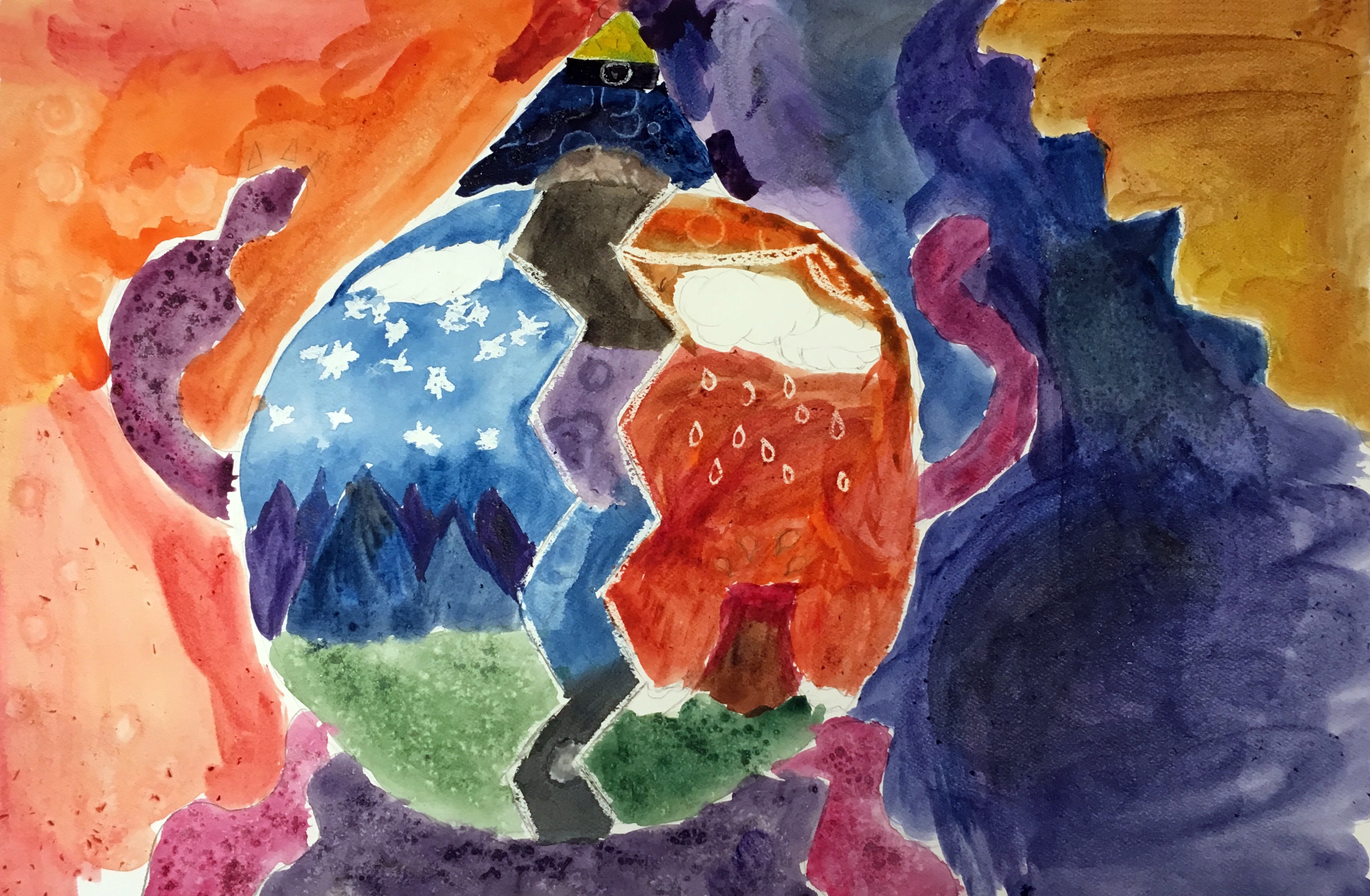The image is an abstract, horizontally rectangular painting that predominantly features a bisected, circular centerpiece. The circle is divided by jagged lines and appears almost like a face, with white clouds suggesting eyes on either side. The left half of the circle depicts a serene, mountainous scene in shades of blue, with falling snow and green ground below, reflecting a calm, possibly nighttime setting. The right half contrasts sharply, showing a fiery, volcanic landscape with a red sky and raindrops, creating a dynamic and intense atmosphere. The triangle above the circle seems to point upwards, with its sections colored in black, blue, and yellow. The background of the image varies from warm tones of orange, red, and yellow on the left to cooler tones of brownish yellows, navy blue, and purples on the right. Additional details include visible brush strokes, possibly suggesting the use of watercolors, and extending purple lines from the central circle, enhancing the painting's intricate and layered appearance. The orange and dark yellow hues towards the right side add depth, completing this visually complex and detailed abstract artwork.